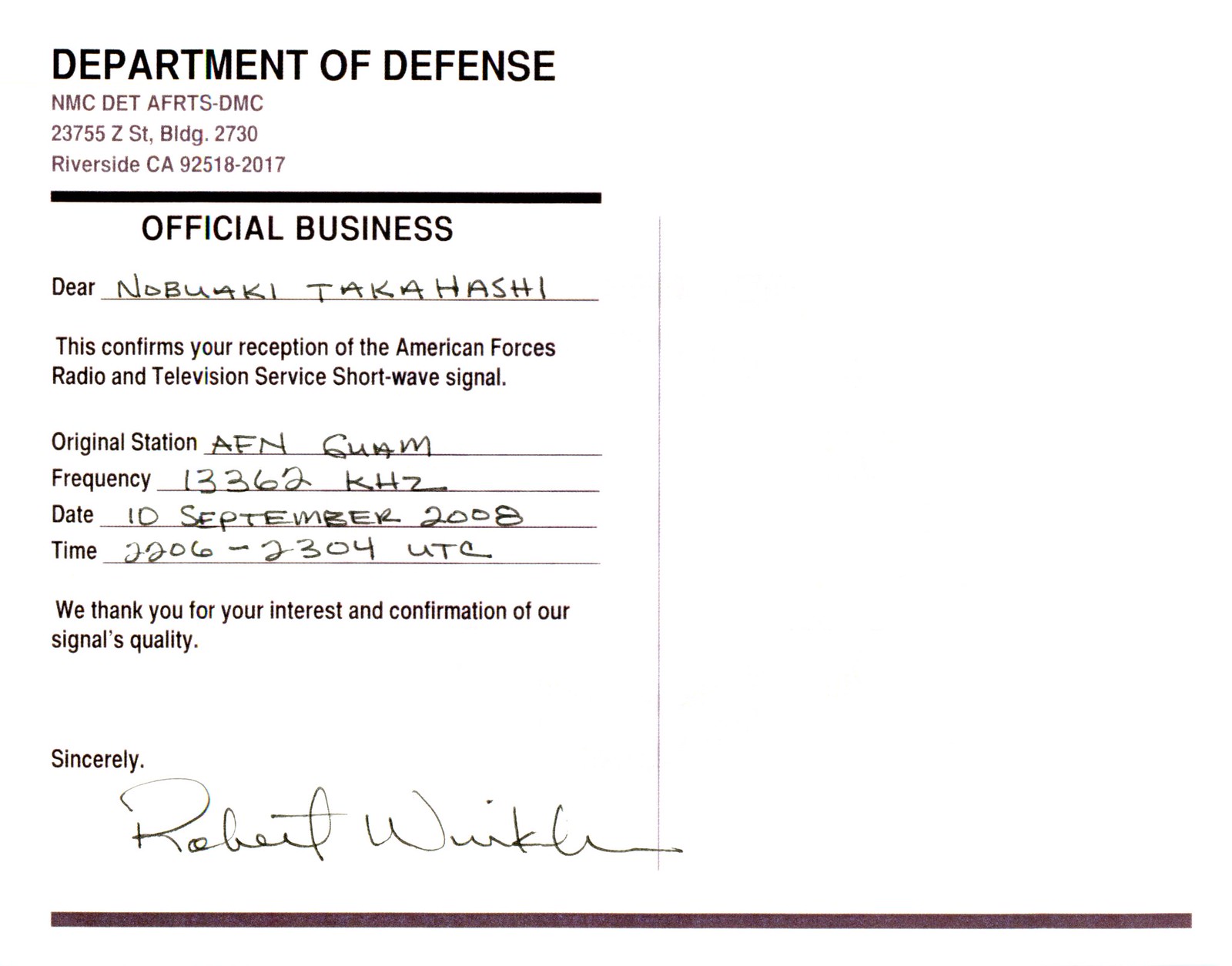The image features a scanned copy of an official document on a white background. The document appears to be a form or certificate from the Department of Defense, with text predominantly in black and some sections in either purple or red. The heading at the top reads "Department of Defense" followed underneath by "NMC DET AFRTS-DMC 23755 ZST BLDG 2730 Riverside CA 92518-2017" in bold. Below this address, a horizontal black line separates it from the main content, which is a letter addressed to Nobuaki Takahashi. The letter confirms the reception of the American Forces Radio and Television Service's shortwave signal from Signal Station AFN Guam on the frequency 13362 KHz, dated 10 September 2008 from 2206-2304 UTC. The letter concludes with a note of gratitude for confirming the signal's quality, signed sincerely, possibly by an individual named Robert Winkler. The right side of the document is entirely blank, emphasizing the text on the left.